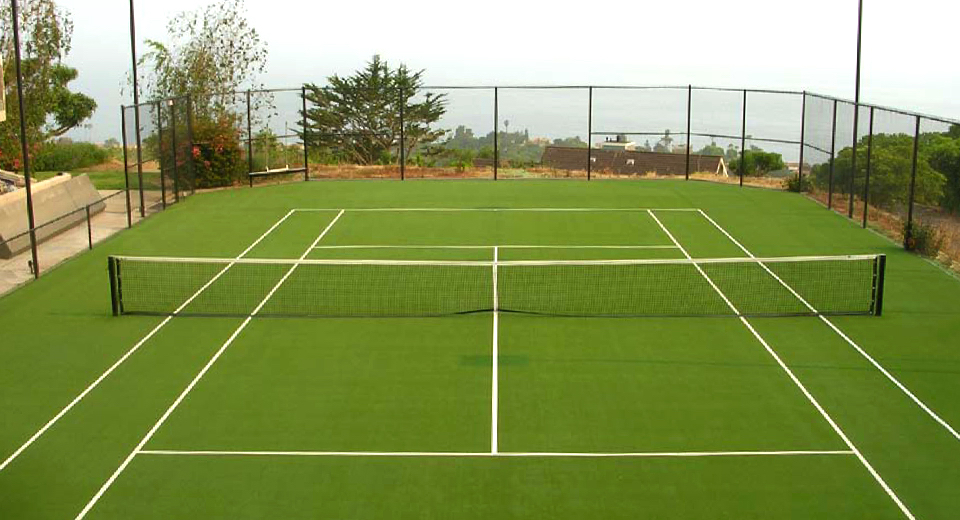The photograph showcases an empty tennis court with vivid, medium to dark green AstroTurf and precisely marked white lines designating the court boundaries. A net spans the center of the court, featuring a black fabric line at the bottom and a white fabric line at the top. The tennis court is surrounded by a six-foot-tall black chain-link fence, providing an enclosed area. On the left side, there is an opening leading out of the court, bordered by a cement wall and sidewalk. 

In the background, above the fence, a hazy, overcast sky merges with the ocean, which appears as a whitish-gray expanse. Several buildings, potentially houses, are situated on the other side of the fence, somewhat downhill from the court. Trees and bushes add a touch of greenery to the surroundings. Additionally, there is a pole on the right side, likely supporting a light for the court. The whole scene gives off an air of serenity, possibly indicative of a country club setting. The photograph is in a horizontal format, enhancing the panoramic view of the entire location.